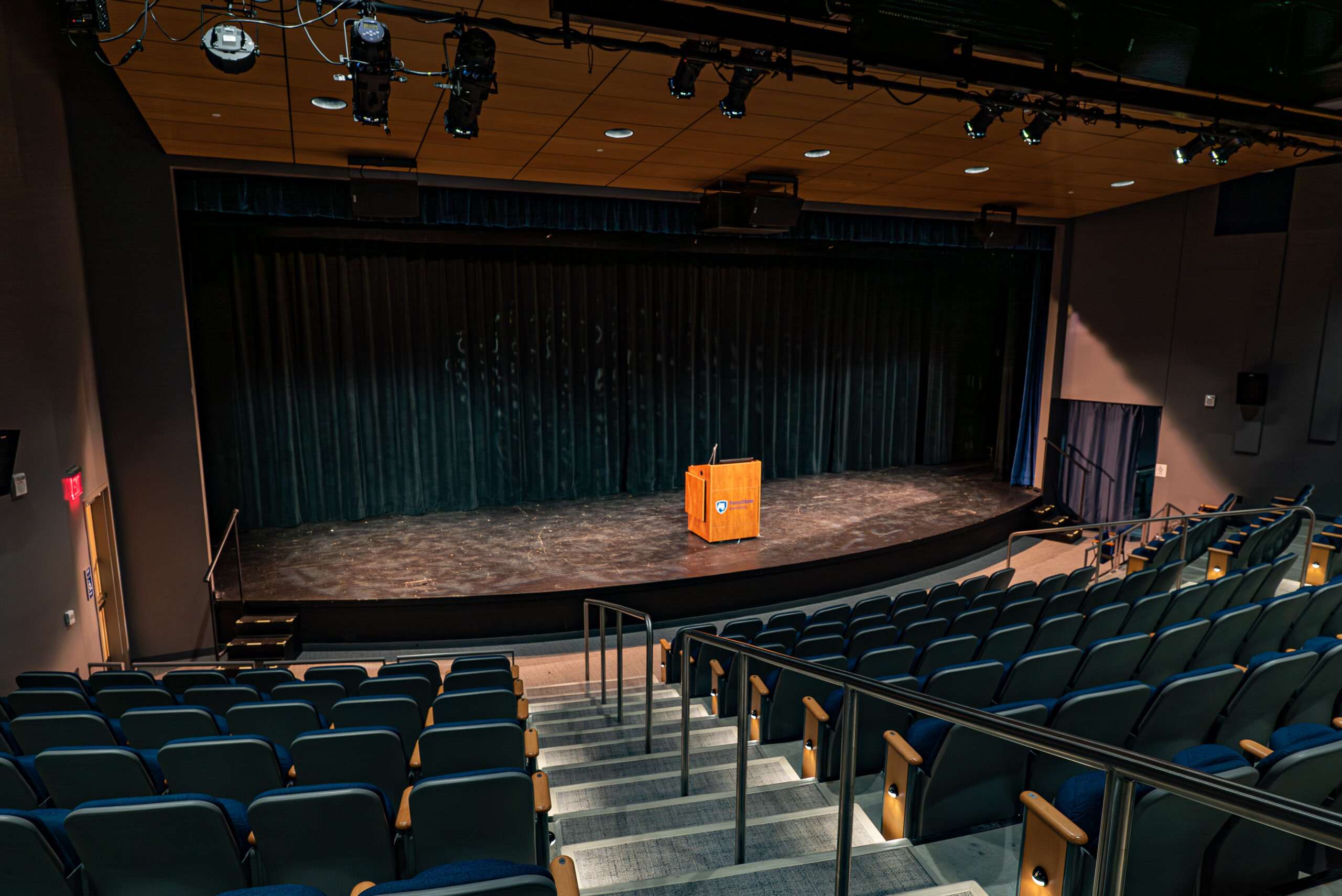The image depicts an auditorium or presentation room, likely within a theater or college environment. The primary focus is on the stage at the front, featuring a golden-brown wooden podium with an emblem and a microphone stand. The stage is framed by dark blue curtains and bordered by black, slightly rounded steps on both the left and right sides. Above the stage, a framework of spotlights is installed in pairs, casting light onto the podium and stage.

In front of the stage, rows of blue chairs with brown wooden armrests and side panels are neatly arranged. The seating area is separated by a gray carpeted staircase running down the center, featuring black metal railings that have a break in one section. To the left side of the image, a wooden door is visible against the brown walls that line both sides of the room. The ceiling above the seating area consists of white square tiles that give off a brownish-yellow hue, complemented by additional lighting. Overall, the room possesses a structured and formal atmosphere, suitable for speeches or educational presentations.